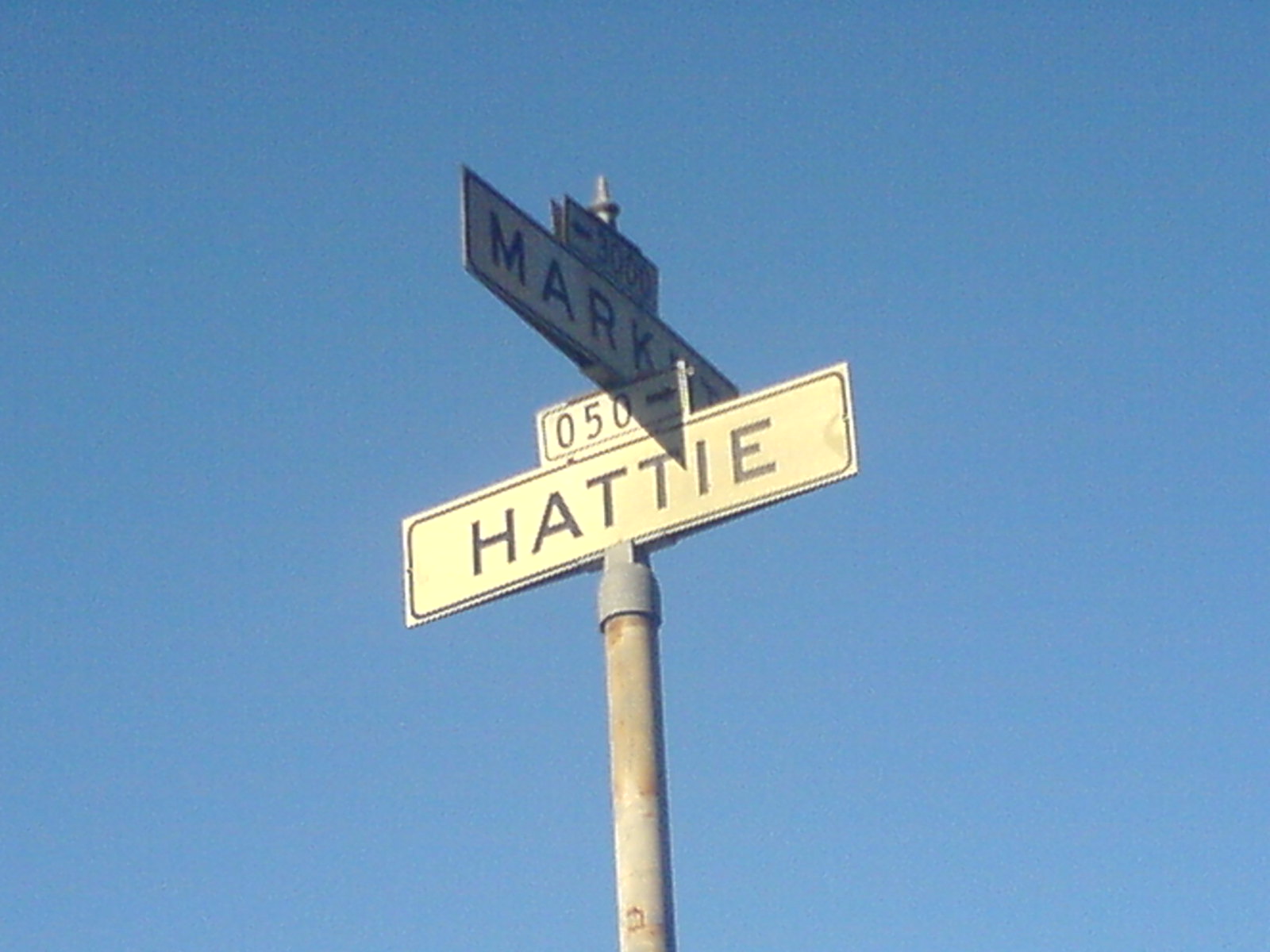The photograph captures a street intersection sign set against a clear, sunny sky with a blue backdrop. The image focuses solely on the intersection sign, which is mounted on a silver metallic pole that shows rust marks in various spots. At the top of the pole, the first sign points towards the top left of the image and appears to read "MARKT," with the letter "E" partially obscured. Just above this sign, a smaller sign shows the number "3000." Below it, a second sign points towards the top right, featuring the number "050" followed by an arrow indicating a rightward direction. Beneath this, another sign reads "Hattie" in black letters. The composition and details of the signs and pole are sharply defined, making them the primary subjects of the photograph.